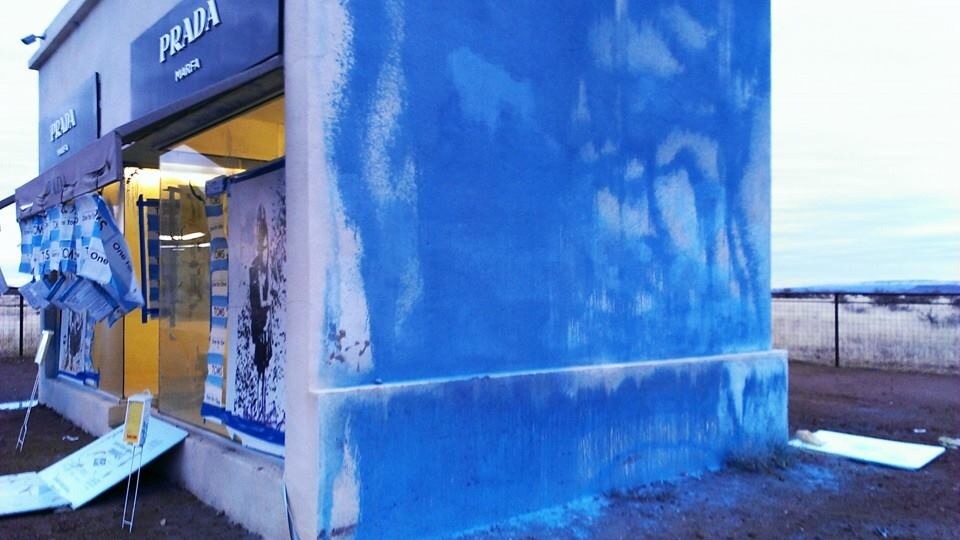This image depicts a solitary, freestanding Prada storefront labeled "Prada Marfa" on two marquee signs atop the entrance. The perspective is mostly from the side, revealing that the building was originally white but has been haphazardly splattered with blue paint, suggesting possible vandalism rather than intentional graffiti. The front of the store features a black awning with a blue and white checkered cloth or flag hanging from one side. In one of the windows, there is a poster of a child. The ground outside is strewn with an assortment of signs and objects. The setting is stark and isolated, with nothing but a fence visible in the background, emphasizing the building's lone presence.